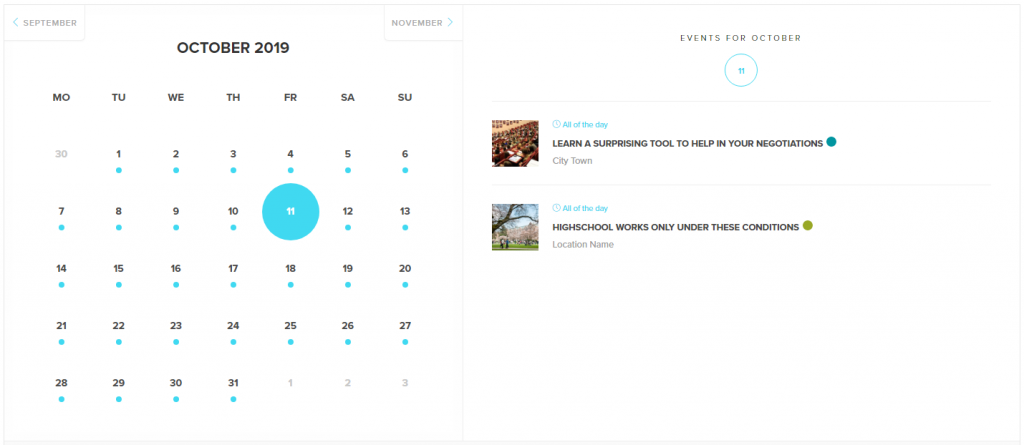The image showcases a website focusing on scheduling, prominently displaying a calendar interface. At the top left, there is a left-pointing arrow next to a box labeled "September." On the right side, there's a similar box labeled "November" with a right-pointing arrow. Centrally placed, in bold text, it reads "October 2019." Below this header, the days of the week are listed from Monday (MO) to Sunday (SU) using their first two letters.

The calendar grid begins with the number "30" in a grayed-out format, followed by numbers arranged sequentially, with each date having a small blue dot below it. The format continues up to the 31st. The numbers for Friday, Saturday, and Sunday (November 1st, 2nd, and 3rd) are light gray, indicating they belong to the following month.

On the right-hand side, there is an additional section titled "Events for October." It features a circular icon with two vertical lines that might represent the number 11. Below this, there are two media thumbnail images with the titles "Learn a Surprising Tool to Help in Your Negotiations" and "High School Works Only Under These Conditions."